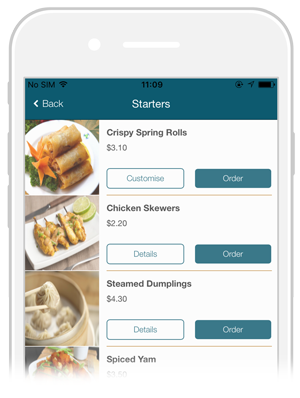The image captures a white cell phone with its screen facing up. In the top left corner of the screen, the status reads "No SIM" alongside a Wi-Fi icon, indicating the device is connected to a wireless network. The top center displays the time as 11:09. On the top right, there is a battery icon showing it is almost fully charged. The top banner of the screen is a grayish blue color. Just below the banner, a white arrow pointing to the left is labeled "Back," while the center text reads "Starters."

The main content of the screen appears to be a webpage displaying menu items, each with a photograph and detailed descriptions.

1. **Crispy Spring Rolls**:
   - A vivid photograph depicts golden brown spring rolls neatly arranged on a white plate. The plate also features a pile of green vegetables topped with sliced carrots.
   - Text reads: "Crispy Spring Rolls - $3.10" accompanied by buttons labeled "Customize" and "Order."

2. **Chicken Skewers**:
   - The image shows several chicken skewers arrayed on a rectangular white plate. Two lime slices are placed at the top-right corner of the plate.
   - Text reads: "Chicken Skewers - $2.20" along with buttons labeled "Details" and "Order."

3. **Steamed Dumplings**:
   - The photograph highlights a beige round container filled with steamed dumplings. A pair of chopsticks, extending from the left edge of the image, is seen holding a dumpling.
   - Text reads: "Steamed Dumplings - $4.30" with buttons labeled "Details" and "Order."

4. **Spiced Yam**:
   - The image shows a white plate piled with spiced yams.
   - Text reads: "Spiced Yam - $3.50."

Each menu item is presented with a high-quality photograph, detailed pricing, and options to customize or order directly.